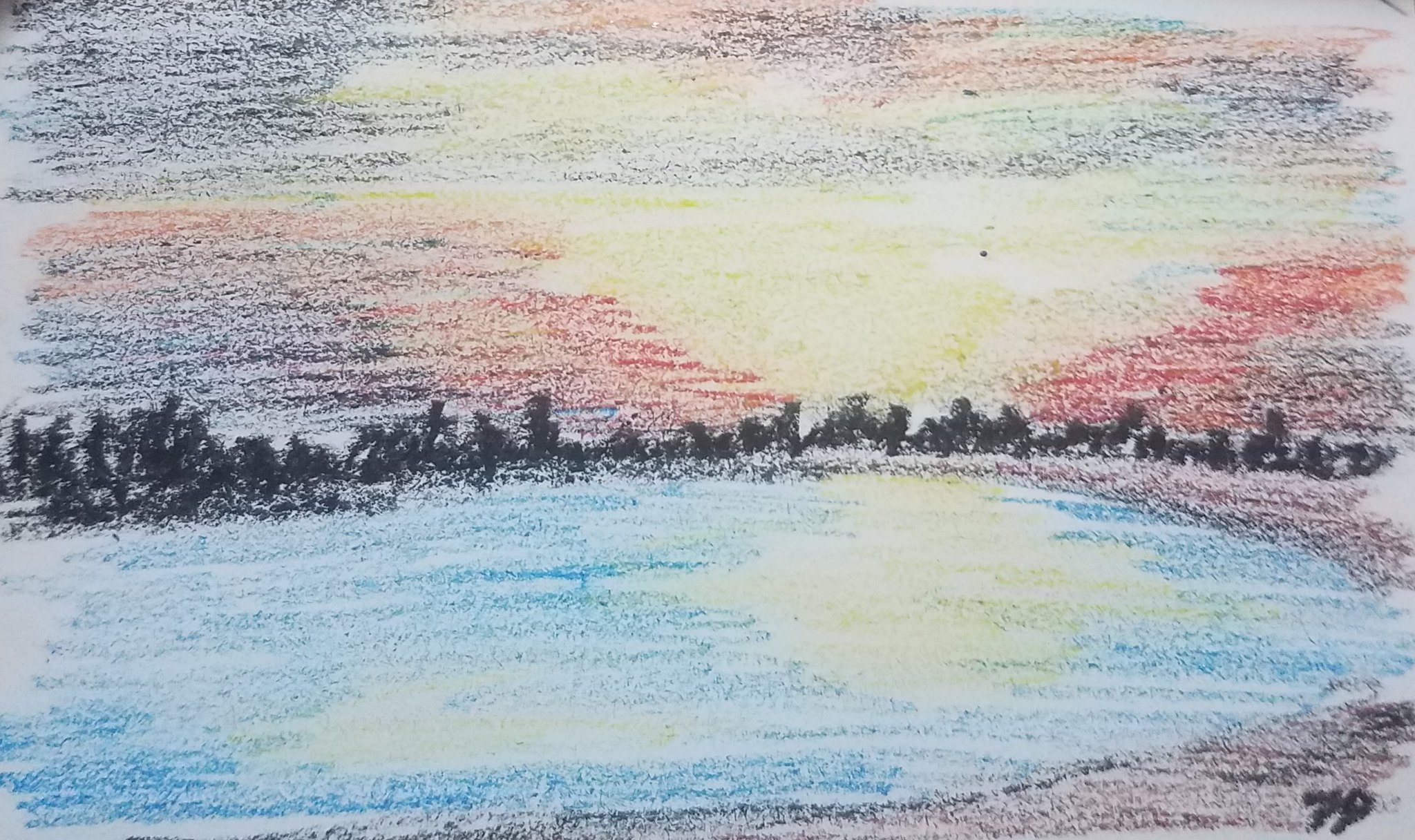This detailed crayon drawing, possibly incorporating pastels, features a tranquil outdoor scene. Dominating the foreground is a large, blue, oval-shaped lake with a distinctive yellow reflection of the sun on its waters, appearing wavy along the edges rather than perfectly mirrored. The shorelines exhibit tones of black and brown, grounding the composition. Beyond the lake, vertical dark black lines suggest a distant tree line on the horizon.

The vibrant sky captures a stunning sunset, with a prominent bright yellow sun ringed by hues of orange, blue, and purple, evoking a sense of layered clouds. The upper half of the image showcases this dynamic sky, blending multiple colors, including patches of red and areas conducive to cloud reflection in the lake below.

The drawing is landscape-oriented and subtly signed in the bottom corner with what appears to be a number—potentially "79" or a slight variation. No people, animals, buildings, or vehicles are depicted, enhancing the serene and undisturbed quality of the lakeside scene. Although the drawing uses a simplistic medium, the blend of colors and attention to detail suggests it might be the work of an impressionist artist rather than a juvenile.